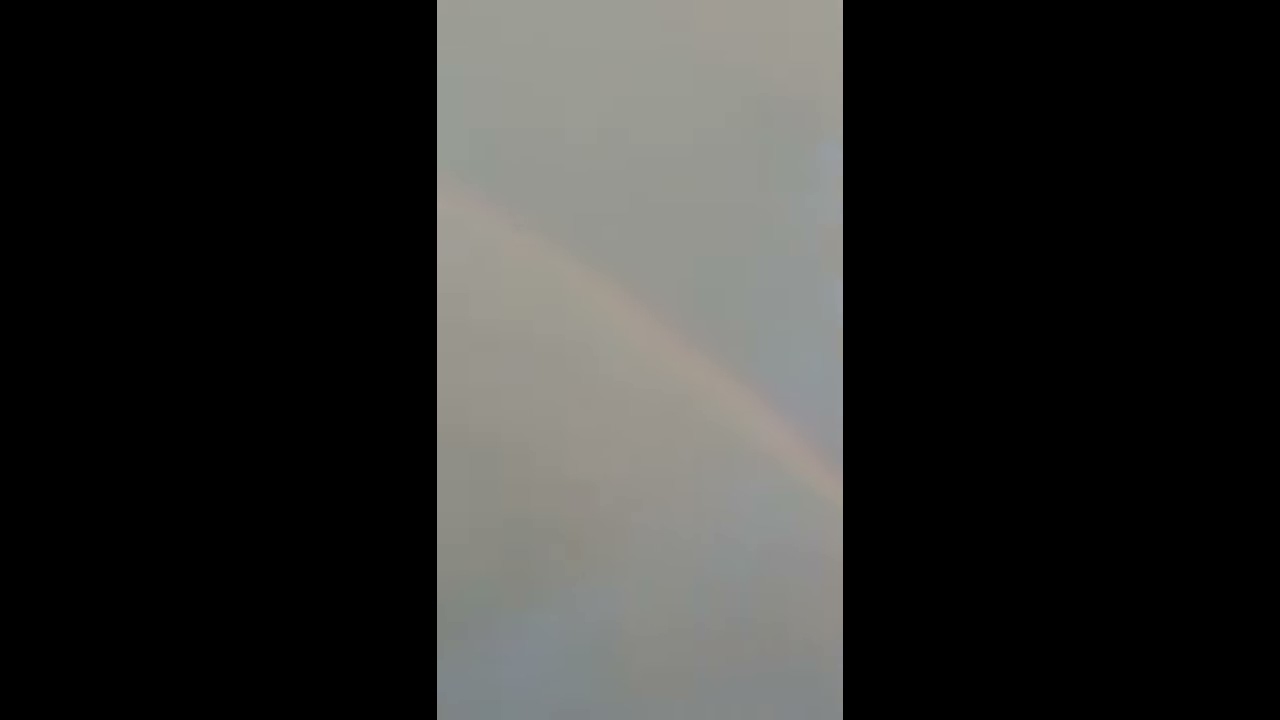In this image, we are presented with a faint rainbow that arcs diagonally from the lower right to the upper left across a hazy, mist-filled sky. The overall scene captures a foggy atmosphere, with the sky displaying a muted palette of light blue and gray tones, indicative of post-storm conditions. The rainbow itself, although weak and slightly blurred, showcases a spectrum of colors, primarily red, yellow, and traces of green. Framing the central foggy scene, where the faint rainbow is the focal point, are two large, solid black rectangular boxes on either side, creating a stark contrast to the misty, gloomy ambiance of the sky. The clarity of the rainbow diminishes within the haziness of the landscape, rendering it an ethereal and fleeting element amidst the soft, foggy backdrop.